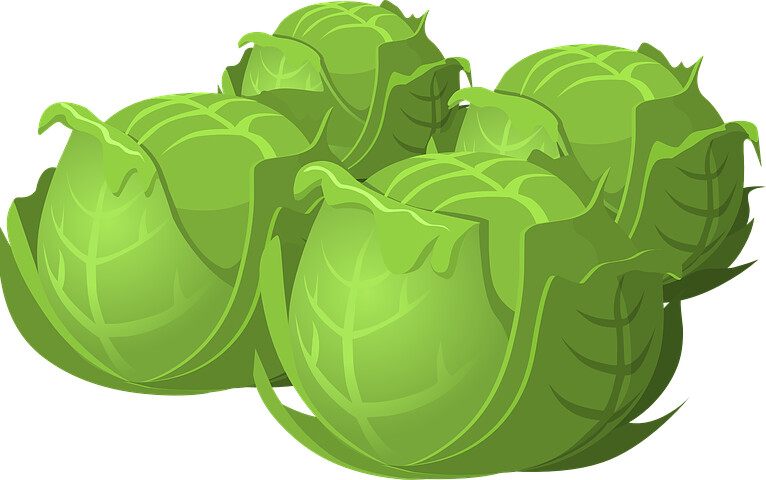This image features an intricately detailed, computer-generated depiction of four cabbage heads against a plain white background. Though resembling real cabbages, they are actually stylized illustrations, potentially crafted by AI or a graphic artist. The cabbages are arranged with one at the front, another slightly behind and to the left, and two more positioned further back, creating a layered effect. Each cabbage showcases well-defined leaf veins and sections, varying in shades of green from bright at the top to darker at the bottom, suggesting depth and shadow. The overall appearance of the cabbages is fresh and vibrant, with a crisp texture that makes them look almost edible despite their digital origin.